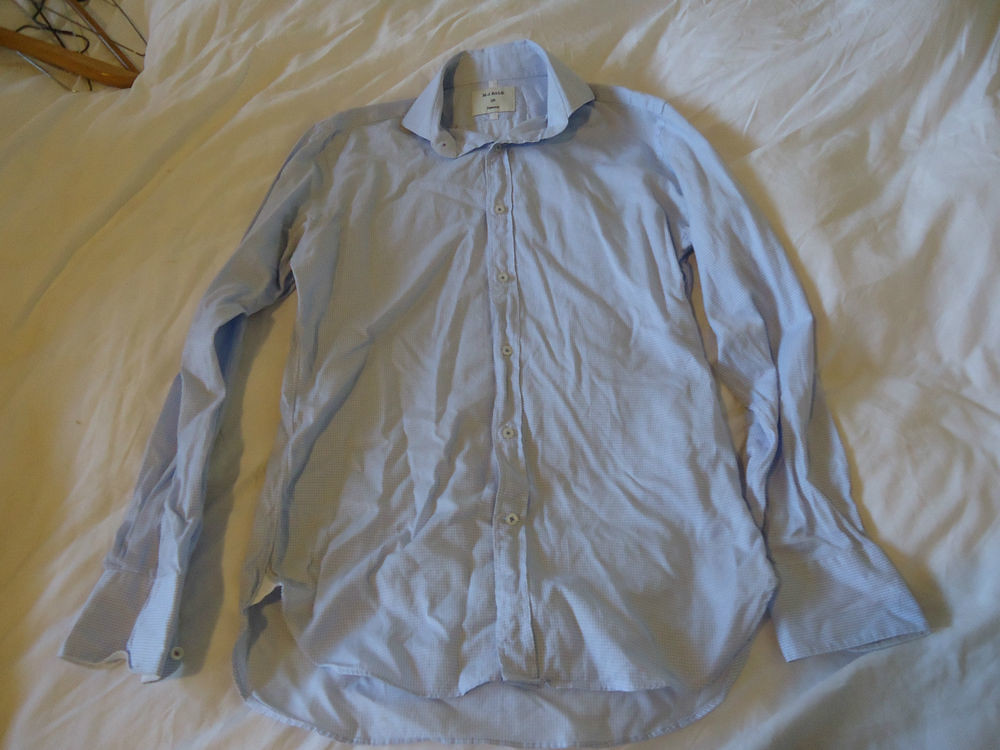The image depicts a light blue, long-sleeve collared shirt, heavily wrinkled, resting on a white, equally wrinkled bed sheet. The shirt, featuring around five or six buttons, has a visible white tag inside, although the brand is indiscernible due to the image's low resolution. In the upper left corner of the image, there is a wooden object draped with a cloth, and some items resembling hangers or wires. Natural light, likely from a window, reflects off both the shirt and the bed sheet, highlighting the wrinkles prominently.